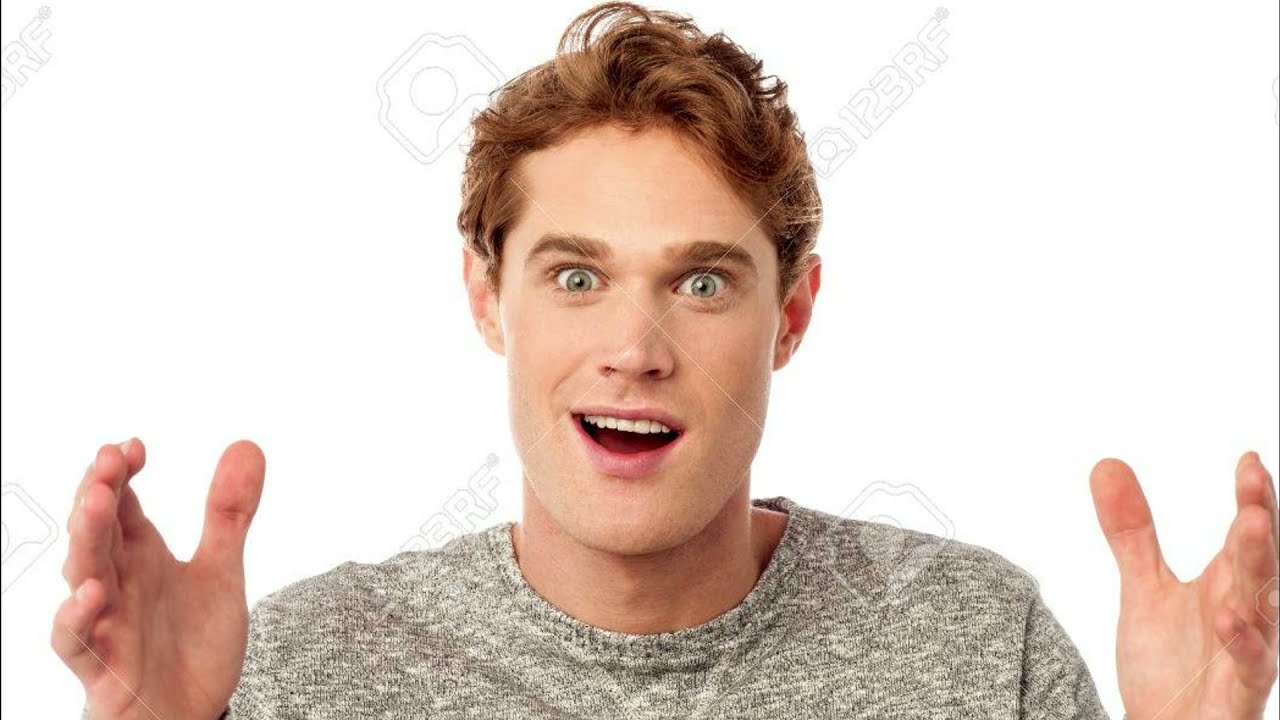The image depicts a young Caucasian man with a bewildered, yet somewhat excited expression. He has medium-length, slightly curly brown hair that twirls to one side, large bushy eyebrows of a similar color, and wide-open light blue eyes. His mouth is agape, revealing his top row of teeth, suggesting a mix of surprise and happiness. He is wearing a gray t-shirt or textured sweater, depending on the interpretation, and his hands are positioned in front of him with palms facing outward, as if emphasizing the width of something. The background is a plain white, prominently marked with a soft gray watermark featuring a small camera icon and the text "123RF," along with an indistinct trademark or copyright symbol. The watermark runs across the entire image, including through the man's face. He occupies nearly the entire frame, with only his upper body visible from the shoulders up.